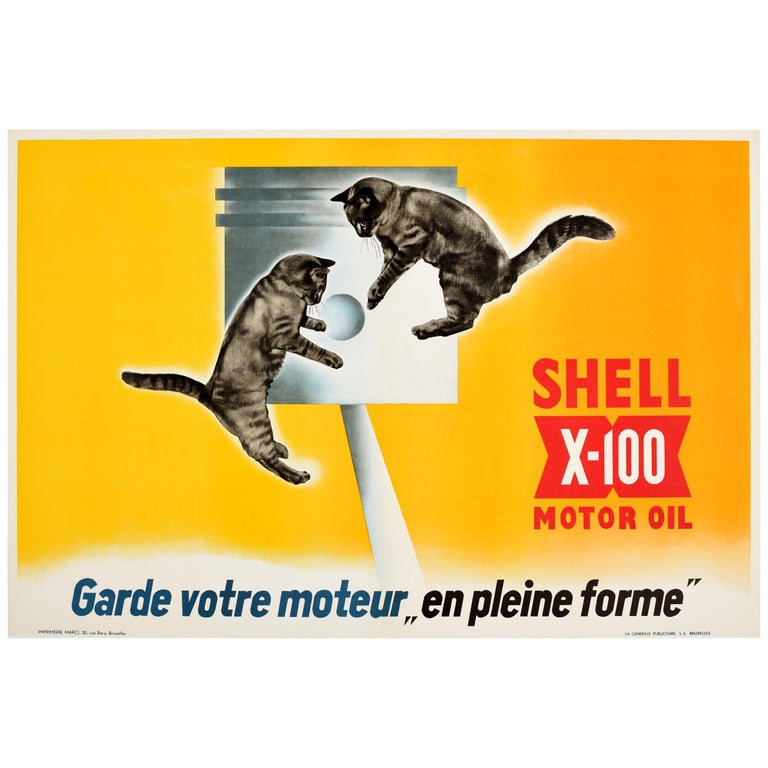This landscape-mode advertisement promotes Shell X100 motor oil, featuring a vibrant orange-yellow gradient background. Dominating the center of the image is a silver piston, around which two cats—gray and black striped tabbies—are playfully leaping in the air. The cats, which add an energetic dynamic to the scene, focus intently on a white ball positioned above them. In the bottom right corner, the iconic red and white Shell X100 motor oil branding stands out. Underneath the image, the French phrase "Garde votre moteur en pleine forme" translates to "Keep your motor in top shape," reinforcing the ad's message.